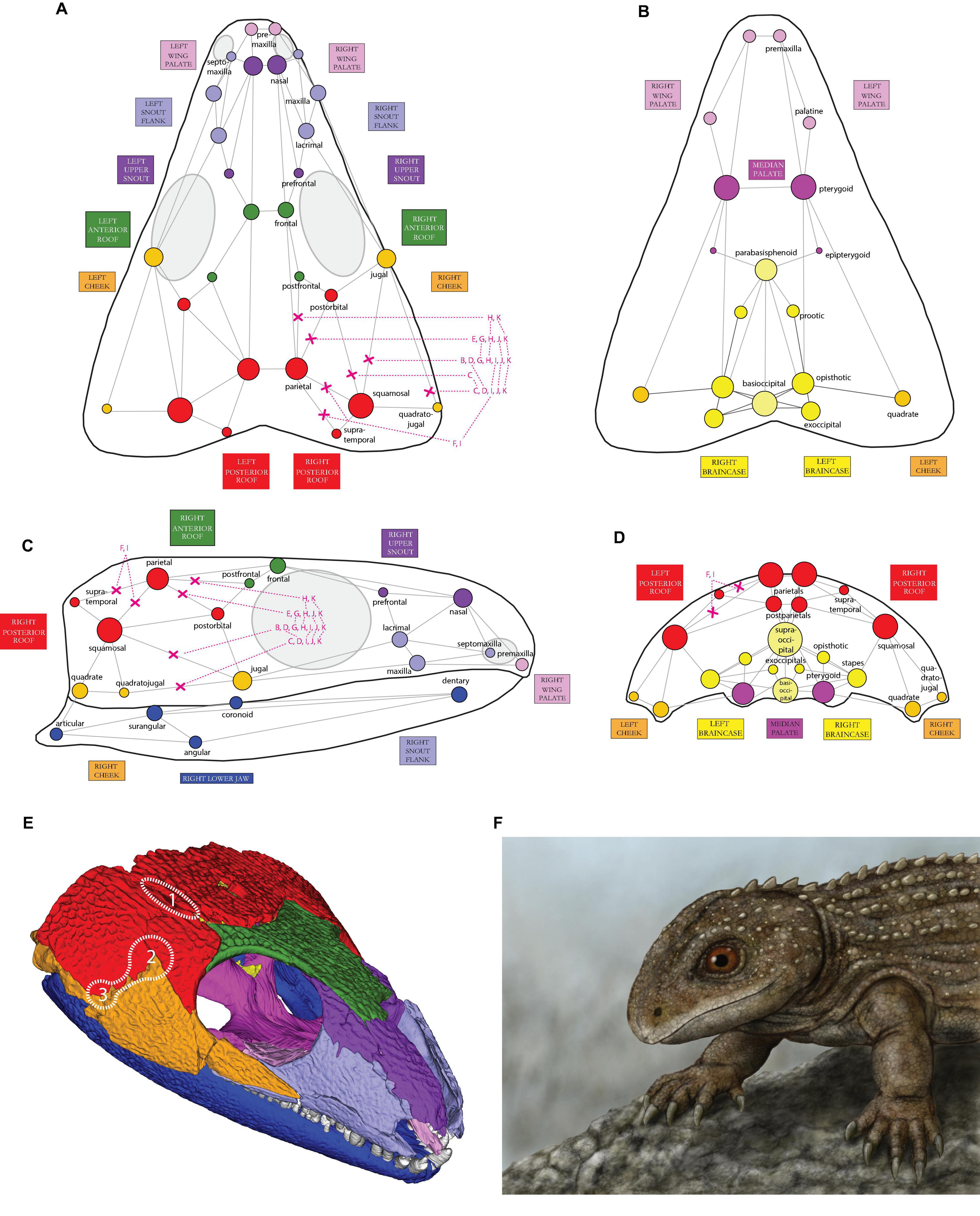The image is a detailed, six-part depiction of a lizard's skull and body. The top row features two overhead views of a lizard skull, outlined in purple, with the nose at the top and the back of the head at the bottom. Both diagrams are annotated with multicolored dots (green, red, yellow, purple) and lines connected to small boxes that describe specific anatomical features. The middle left image displays a side view of the skull, showing the nose on the right and the back of the head on the left, along with an outline of the eyeball and mouth. This side view also includes red, green, purple, blue, and yellow dots, each linked to descriptive annotations. The middle right image presents a view of the top cranium with similar color-coded dots and explanatory boxes. In the bottom left, a vividly painted representation of the lizard's skull highlights various parts in different colors: green over the eyes, red atop the skull, orange along the jawline, blue under the jaw, purple down the nose and around the eyes, and light blue on the sides of the nose. The final picture in the bottom right corner portrays a computer-generated, lifelike drawing of the lizard, showing its light green, scaled body with its front legs and head visible, facing left, and standing on a rock.